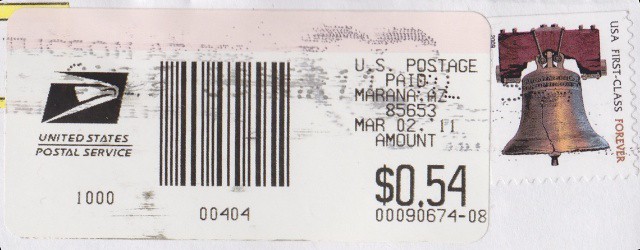The image features a postal label and a postal stamp intricately detailed with various inscriptions and logos. The postal label prominently displays the logo of the United States Postal Service, followed by the name in all capital letters separated by a black horizontal line. Below this line, the number "1000" is clearly visible. 

In the upper left corner of the label, there's a stamped mark indicating "Tucson, AZ," accompanied by several other printed details that are difficult to decipher. To the right of this, a heart shape prominently features a barcode with the number "00404." Below it, the label lists:

- U.S. Postage
- Paid
- Marina, AZ 85653
- Mar 02, 11 (indicating the date March 2nd, 2011)
- A mail fee of $0.54
- The tracking number "0090674-08"

Adjacent to the barcode, the postal stamp depicts a cracked bell supported by a reddish-colored stand. To the right of this image, it reads "U.S. First-Class Forever." The words "U.S. First-Class" are in black, while "Forever" is in a lighter red hue with white shading, giving the lettering a distinct appearance.